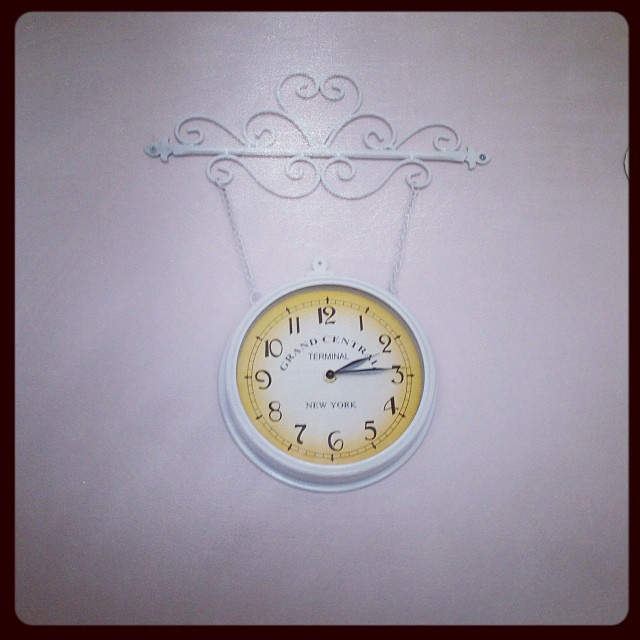This image depicts a unique clock adorned with an ornate suspension system. The clock is connected to an intricate rod featuring swirling patterns at the top and bottom and is held in place by chains on either side. The clock itself is round with a white frame and features a yellow border with a white face. Black numerals in a counterclockwise arrangement mark the hours, and matching black hands indicate the time. At the center of the clock face, the words "Grand Central" are prominently displayed, with "Terminal" positioned just below. The elegant design and reverse numbering give the clock a distinctive and eye-catching appearance.